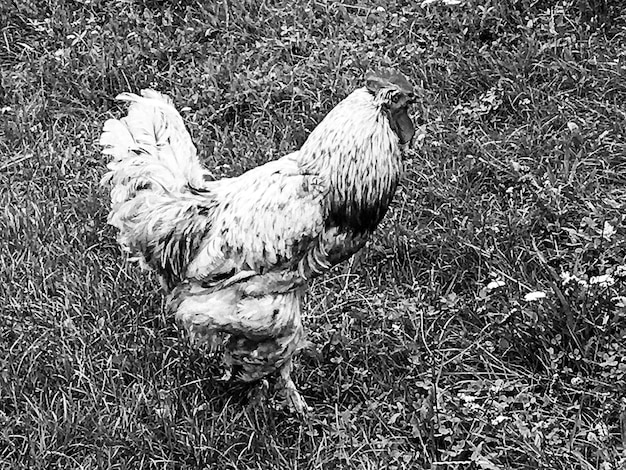This horizontally-aligned, rectangular black-and-white photograph captures a grainy and slightly blurry side view of a rooster standing in an ankle-high grassy field. The rooster, primarily white in color with a darker patch on its underside, is facing towards the right side of the image. Noticeable details include its small head adorned with a comb and wattle, and large feathers pointing upwards. The grassy field is dotted with some white wildflowers, particularly visible in a patch on the right side of the image. There are no other animals or objects in the picture, nor any borders or text around it. The overall coloration appears brownish due to the black-and-white nature of the photograph, adding an aged feel to the scene.